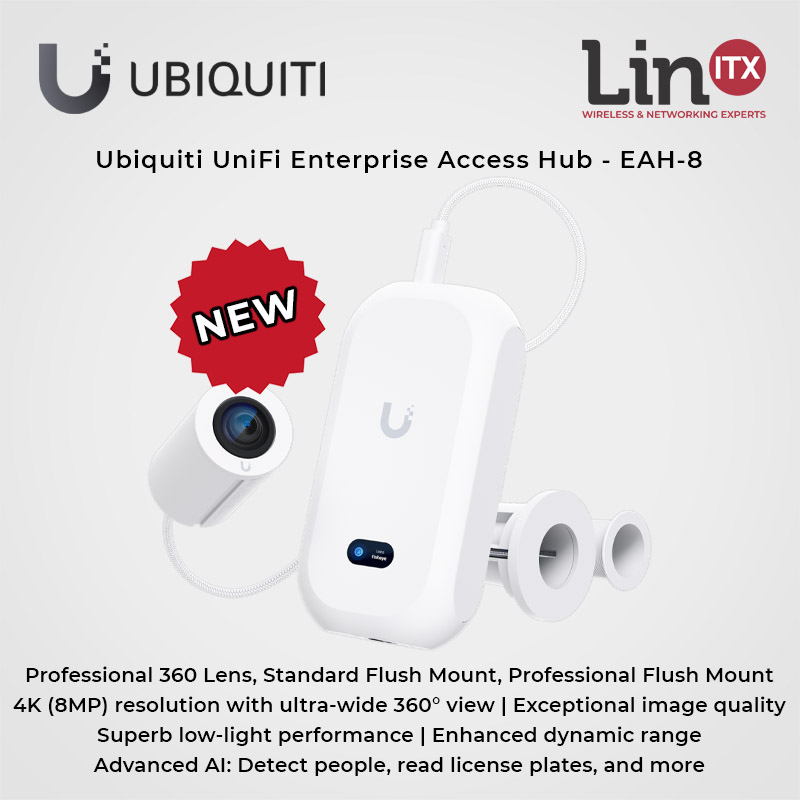This is an advertisement for the Ubiquiti Unify Enterprise Access Hub EAH8, presented by Lin ITX Wireless and Networking Experts. The ad features a prominent image of the product, a white AI camera, potentially a dash cam, against a slightly grayish white background, which makes the camera stand out. The camera has a large main component with a wire extending from it that connects to the camera lens. At the top of the ad, there is a noticeable red sticker labeled "new" in white letters. The detailed specifications listed below highlight the camera’s features: a professional 360-degree lens with both standard and professional flush mounts, 4K 8MP resolution providing an ultra-wide 360-degree view, exceptional image quality with superb low-light performance, enhanced dynamic range, and advanced AI capabilities that can detect people, read license plates, and more.